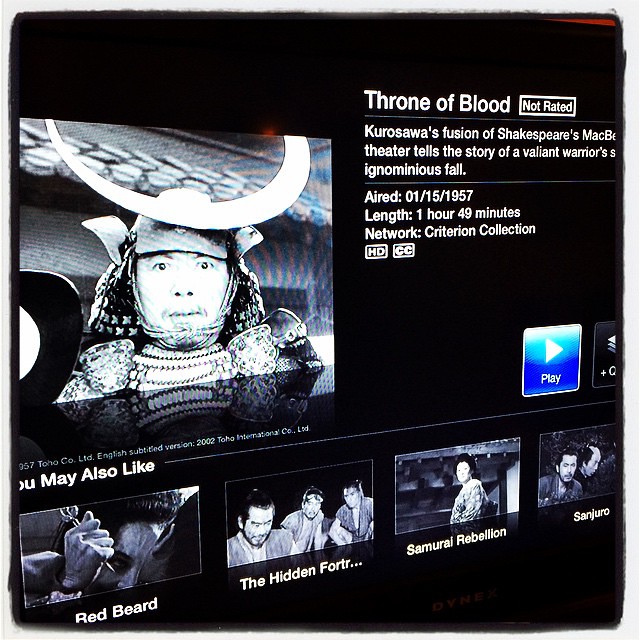This image captures a photograph of a TV screen displaying a movie selection interface on a streaming platform. The focal point is a black-and-white portrait of an Asian male warrior clad in ornate metal armor and a detailed helmet with a large horn, standing in front of an Asian building. To the right of the photograph, text reads "Throne of Blood," marked as "Not Rated." Below, a description elaborates: "Kurosawa's fusion of Shakespeare's Macbeth tells the story of a valiant warrior's ignominious fall." Additional details include the air date "01-15-1957" and the runtime "1 hour 49 minutes" under the Criterion Collection. There's a play button prominent on the lower right, and beneath it, the section "You May Also Like" showcases four other black-and-white still images of suggested movies. The layout is a harmonious blend of black-and-white photography, graphic design, and informative typography.